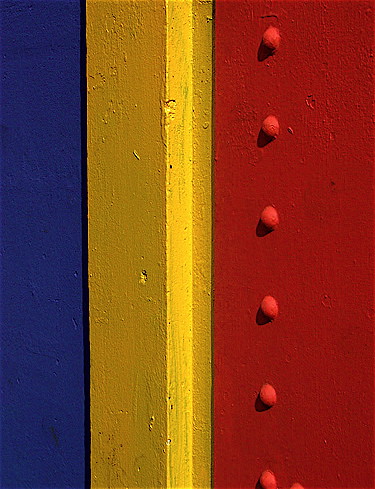This full-color outdoor photograph captures three vertical rectangular panels, each of a different width but identical height, aligned side by side. From left to right, the first panel is blue. The second, yellow panel in the middle, features an intricate crevice design, creating a play of light and shadow that gives it a unique texture. The third panel on the far right is red, marked by a series of evenly spaced, raised red dots resembling rivets that run vertically through the center of the panel. The lighting hits the panels in such a way that it accentuates the different colors and textures, adding depth and dimension to their appearance.